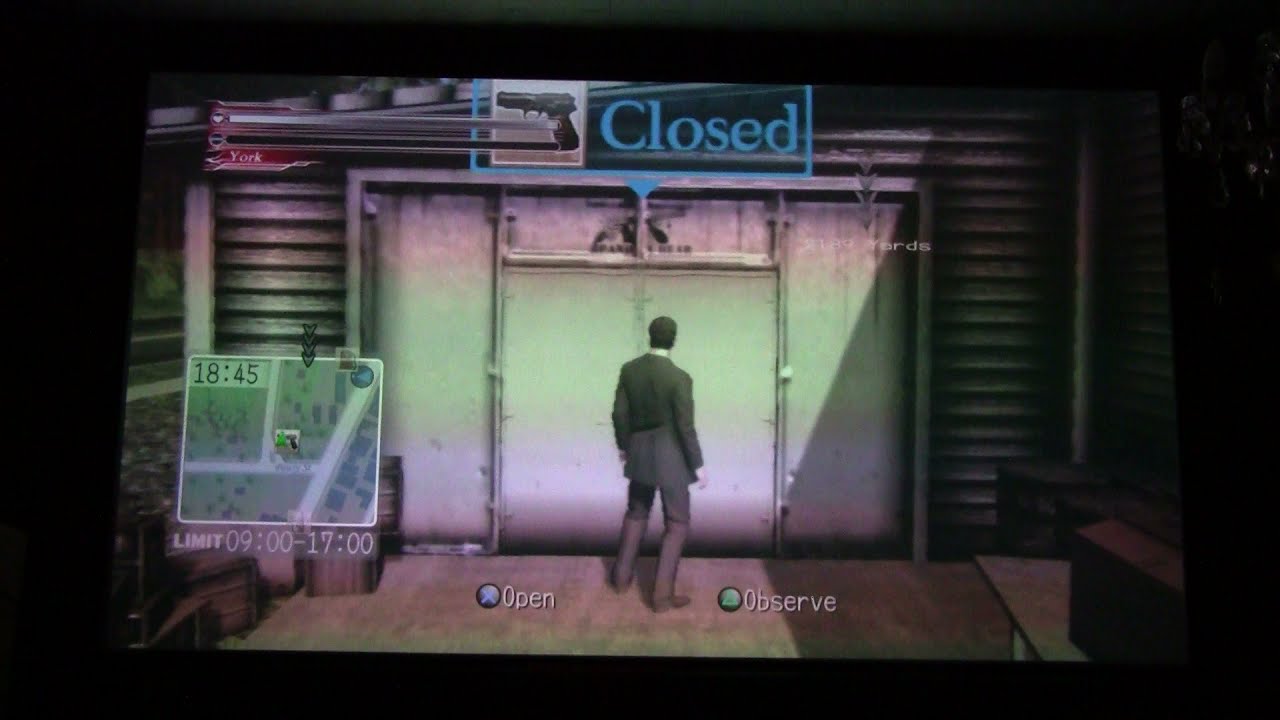This horizontal rectangular image is a snapshot from a video game, presenting a scene framed by a solid black border. At the top of the screen, there is a small icon of a handgun pointing left, accompanied by the word "CLOSED" in blue letters. Below this, a man stands with his back to the viewer, dressed in a grayish-brown suit with a white-collared shirt, his short brown hair visible. He is positioned in front of what appears to be a gray stone or industrial tin double door, resembling a garage door that might raise up. The door has white stripes across it, giving it an industrial look.

The setting seems to be either a warehouse or factory, with a grayish white stone wall and semantic ground around. To his left, the screen shows a square informational area containing a map, indicating his location in relation to roads and blocks within the game's environment. The map also displays the time "18:45" along with various other numbers. Towards the bottom left of the screen are the options "OPEN" and "OBSERVE," suggesting possible actions for the player, further emphasizing the interactive nature of the scene. Additionally, there are boxes laid out near the man, potentially indicating the room's industrial context.